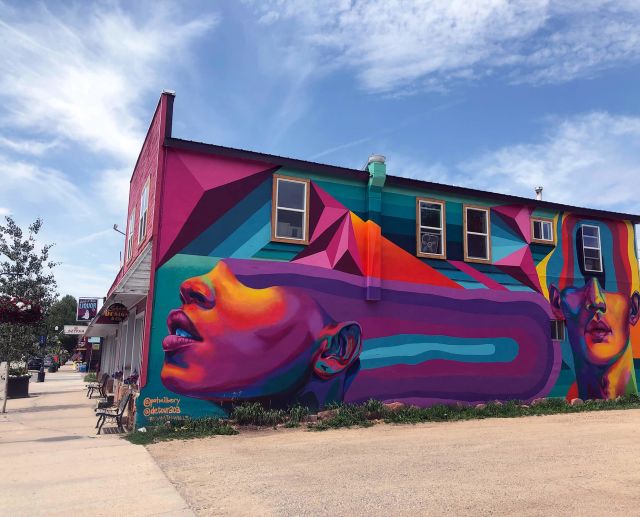The image depicts a brightly painted, two-story rectangular building, likely situated in a suburban town center. The lower level appears to house a business, identifiable by the benches, potted plants, and sidewalk in front, while the upper level features five windows but lacks any sort of commercial signage. The most striking aspect of the building is an expansive mural that blankets the entire visible side wall, rendered in vivid, almost surreal colors. The mural is dominated by the lower faces of a man and a woman—the woman's face is turned to the left with her lips pointing towards the front of the building, while the man's face, located at the far right, faces into an adjacent parking lot. 

The woman's face is accentuated with full lips and a dark complexion, and where her eyes should be, two purple streaks—one light and one dark—extend backwards and curve downwards. Additional blue streaks, both light and dark, emanate from her ear. The man’s face, light-skinned, features a striking pattern of red, yellow, and purple streaks radiating from his eyes upwards, resembling a colorful, abstract rainbow. Both faces are set against a pink-purplish backdrop interspersed with blue and decorated with small purple triangles, blending the figures and their abstract elements into a cohesive artistic composition. The mural is an intricate palette of oranges, pinks, purples, aqua, turquoise, blue, yellow, and reds, creating a captivating visual that draws the eye amidst the surrounding landscaping, trees, and other nearby buildings.